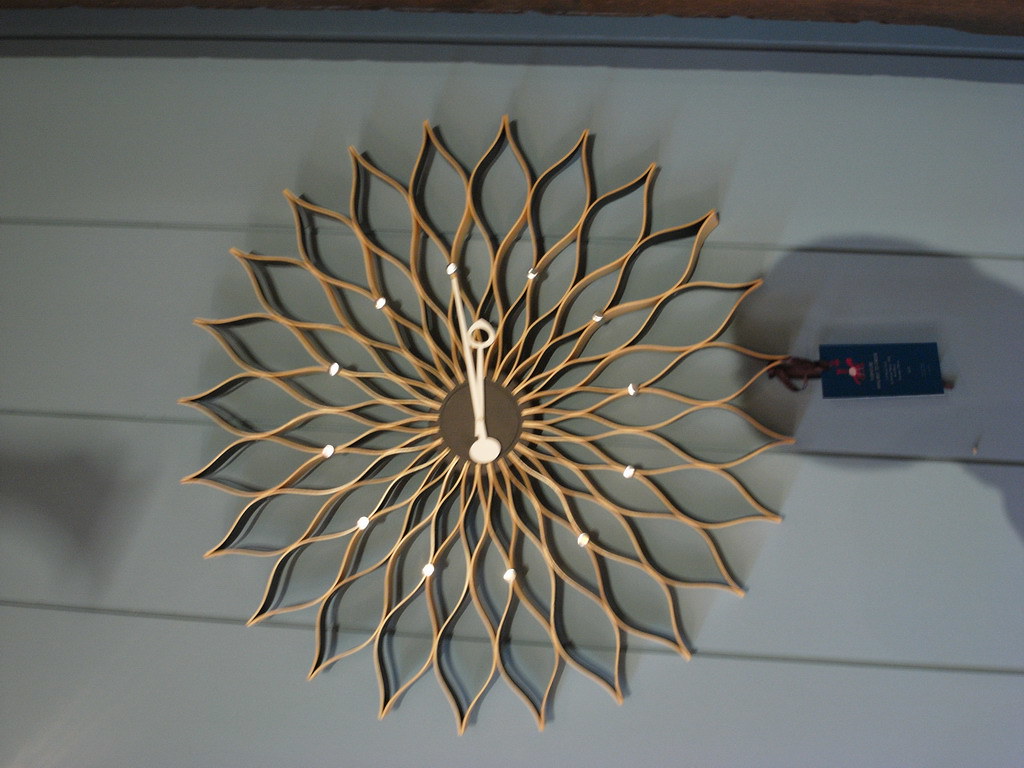The image displays an elaborate and decorative clock mounted on what appears to be the white or off-white vertical paneling of a house exterior, characterized by visible grooves between the wooden slats. The clock is intricate, resembling a gold-colored sunburst or flower design, with multiple layers of metal petals radiating outward. These petals form four concentric circles of curved diamond shapes, each larger as they extend outward. There are no traditional numbers on this clock; instead, there are 12 small, reflective dots or balls marking the hours.

At the core of the clock is a brown circular center, from which two gold-colored hands—a long minute hand, a shorter hour hand, and a straightforward second hand—radiate, showing a time of 11:55. The hands are detailed, with one featuring an oval and another a circular, possibly pointed end. The entire clock face lacks a protective glass covering, allowing the metal sun rays and petals to reflect the light and casting intricate shadows.

A black tag or label with writing remains attached to the clock, hinting it might be brand new. The shadows from the photographer's arm and an unidentified object further enrich the texture of the scene. To the right, there appears to be a power source, possibly providing energy to the clock and its luminous features.